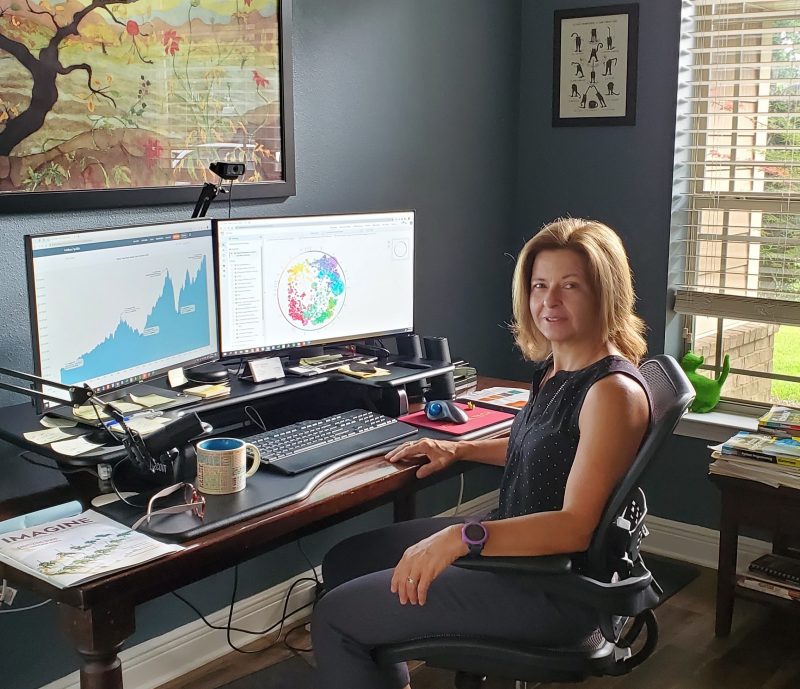A blonde woman with shoulder-length hair is sitting at a wooden desk in a home office, smiling at the camera. She is dressed in a black sleeveless shirt and black pants, accessorized with a black watch featuring a purple face on her left wrist and a wedding ring. The desk is arranged with two monitors: the left one displays a blue graph while the right one shows a colorful circular chart. Her workspace is organized with essential items like a computer mouse, a keyboard, a coffee mug, and numerous sticky notes. 

In the background, the walls are painted a darker blue, and there is a window adorned with pulled-up blinds, revealing a small green cat statue on the windowsill. A stack of books is visible on a small table beneath the window. Above the monitors, two pictures are mounted on the wall, one of which appears to be a Japanese-style painting featuring trees and plants. The woman is seated in an office chair, turning slightly to face the camera, radiating a pleasant and welcoming demeanor.